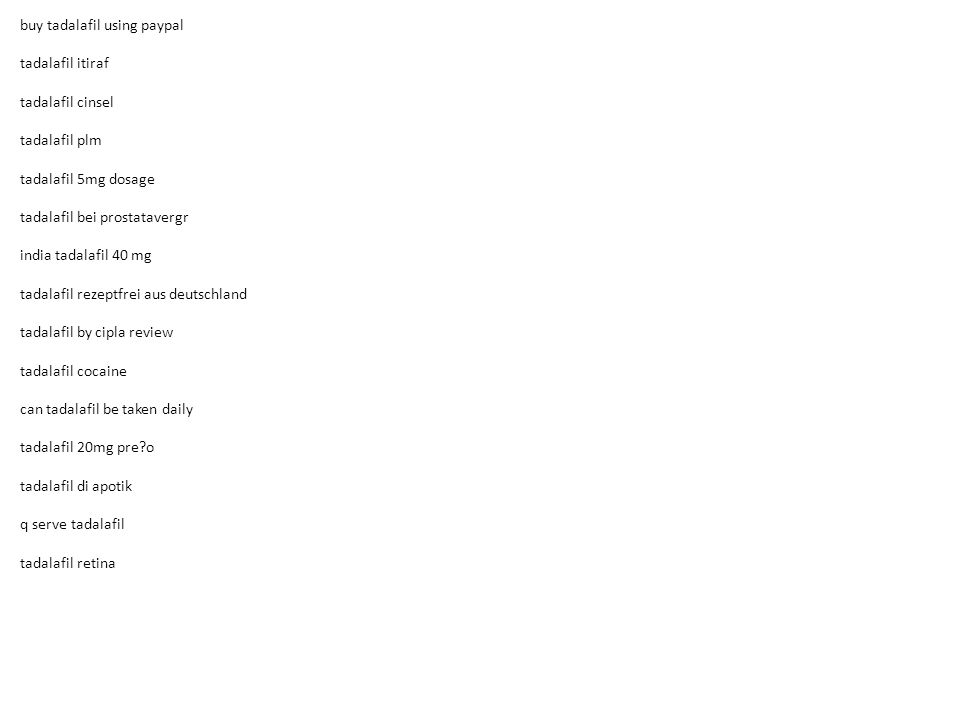In this image, set against a stark white background that occupies approximately three-fourths of the space, there is a list of text in small, black, lowercase font located in the upper left quadrant. The text appears to be a compilation of various phrases related to "Tetalafil," a term repeated prominently throughout. The list includes the following entries: "buy tetalafil using PayPal," "tetalafil Iteraf," "tetalafil Sinsul," "tetalafil PLM," "tetalafil 5 milligram dosage," "tetalafil Bay Prostata Verger," "India tetalafil 40 milligram," "tetalafil Rezept Fry Aus Deutschland," "tetalafil by Cipla Review," "tetalafil Cocaine," "can tetalafil be taken daily?" "tetalafil 20 mg," "tetalafil D Apotic," "Q-Serve tetalafil," and "tetalafil Retina." The minimalistic and clinically-focused layout emphasizes the overwhelming presence of the term "Tetalafil," suggesting a comprehensive list of its types, uses, dosages, and related queries.